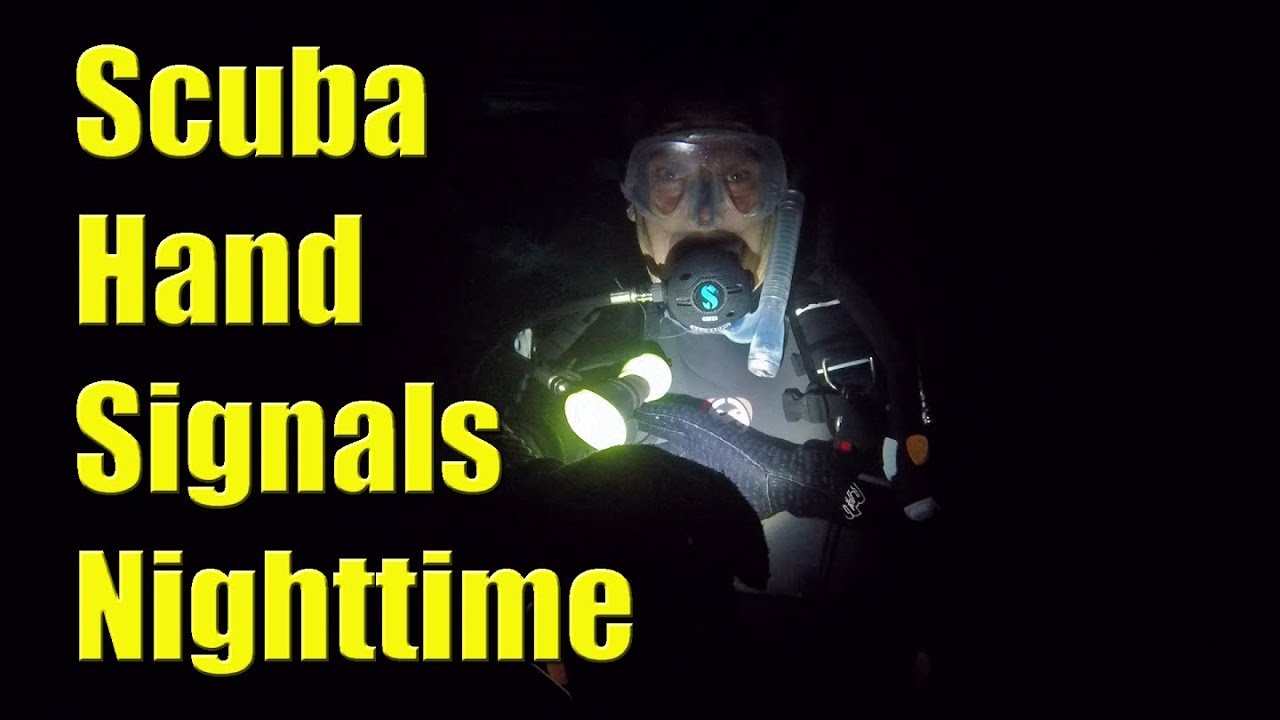The photograph captures a scuba diver submerged in pitch-black water, with a flashlight illuminating only him against the opaque background. Bold, yellow text on the left side of the image reads "Scuba Hand Signals Nighttime." The man, donned in full scuba gear including a mask, goggles, a black wetsuit, gloves with white designs, and a breathing apparatus with an 'S' insignia on it, is staring intently at the camera, exuding a serious demeanor. His flashlight pierces the darkness, revealing no details of his surroundings, emphasizing the isolation and potential danger of the underwater environment.